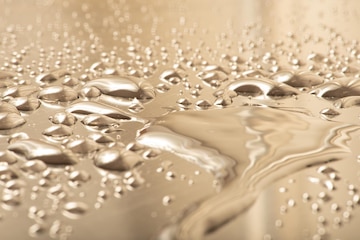The image is a detailed close-up of a brownish-bronze surface with a metallic sheen, reminiscent of molten liquid or a fluid metal. The surface, exhibiting a sandy opalescent gold appearance with varying shades of metallic whites and silvers, is covered in numerous water-like droplets that range in size. Some droplets are large and rectangular, while others are tiny, forming a pattern across the entire image. There are notable groupings of larger bubbles on both the left and right sides. The center of the image features a small, flat pool or valley, giving the impression of flowing liquid with raised, ridged areas around it. The detailed texture and bubble distribution suggest a dynamic, possibly bubbling surface, enhancing the image's liquid-like aesthetics without any text or identifying markers.